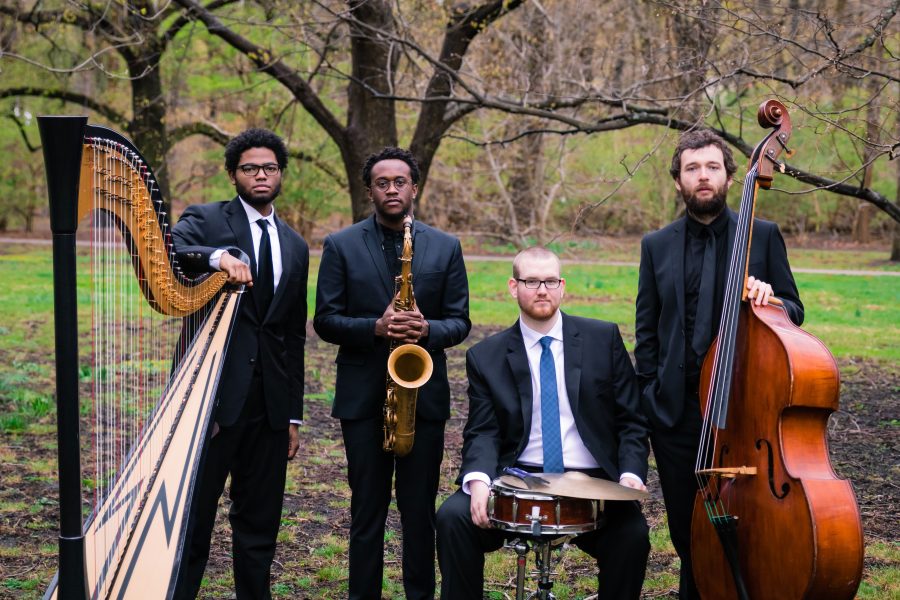In a serene, grassy natural area with trees in the background, four young men, seemingly aged between 19 and 26, pose for the camera in dark-colored suits, suggesting a musical ensemble. The two men on the left are Black; the far-left man stands behind a giant harp, wearing a white shirt with a black tie, while the man next to him holds a saxophone, dressed similarly. The third man, seated in front of a drum set and cymbal, is Caucasian and sports a white shirt with a blue tie. The man on the right, also Caucasian with a beard, holds a cello, completing the quartet. The outdoor setting and formal attire imply they are preparing for a performance, juxtaposed against the natural backdrop.